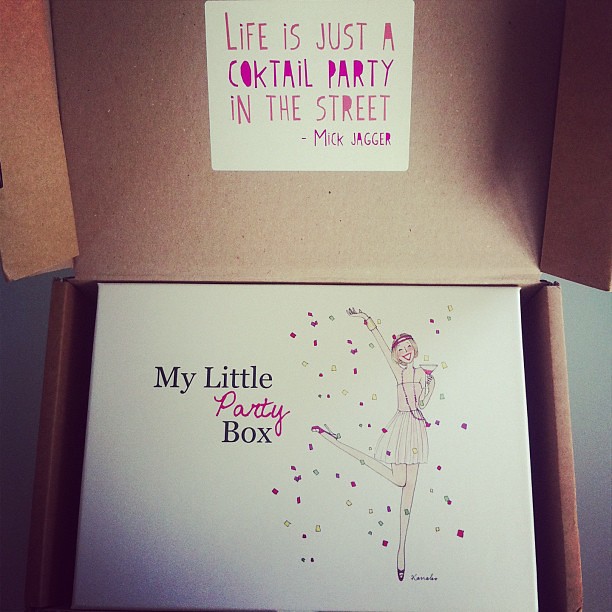The image depicts an unboxing scene where a larger brown cardboard box, opened to reveal its contents, contains a smaller white box inside. The lid of the larger box is lifted, showcasing a colorful, party-like quote in red and pink stylized lettering that reads, "Life is just a cocktail party in the street, Mick Jagger." Notably, the word "cocktail" is misspelled as "C-O-K-T-A-I-L," with the interior letters artfully colored pink. Nestled within is a pristine white box labeled "my little party box" in a mix of typical black and cursive red lettering. The focal point of this smaller box is an illustration of a jubilant woman in a pink party dress, complete with a necklace and headband. She's holding a martini glass aloft in one hand, the other hand thrown back, and her left leg playfully bent, all amidst a shower of confetti. The artwork exudes a celebratory mood, perfectly complementing the festive theme set by the larger box's quote.